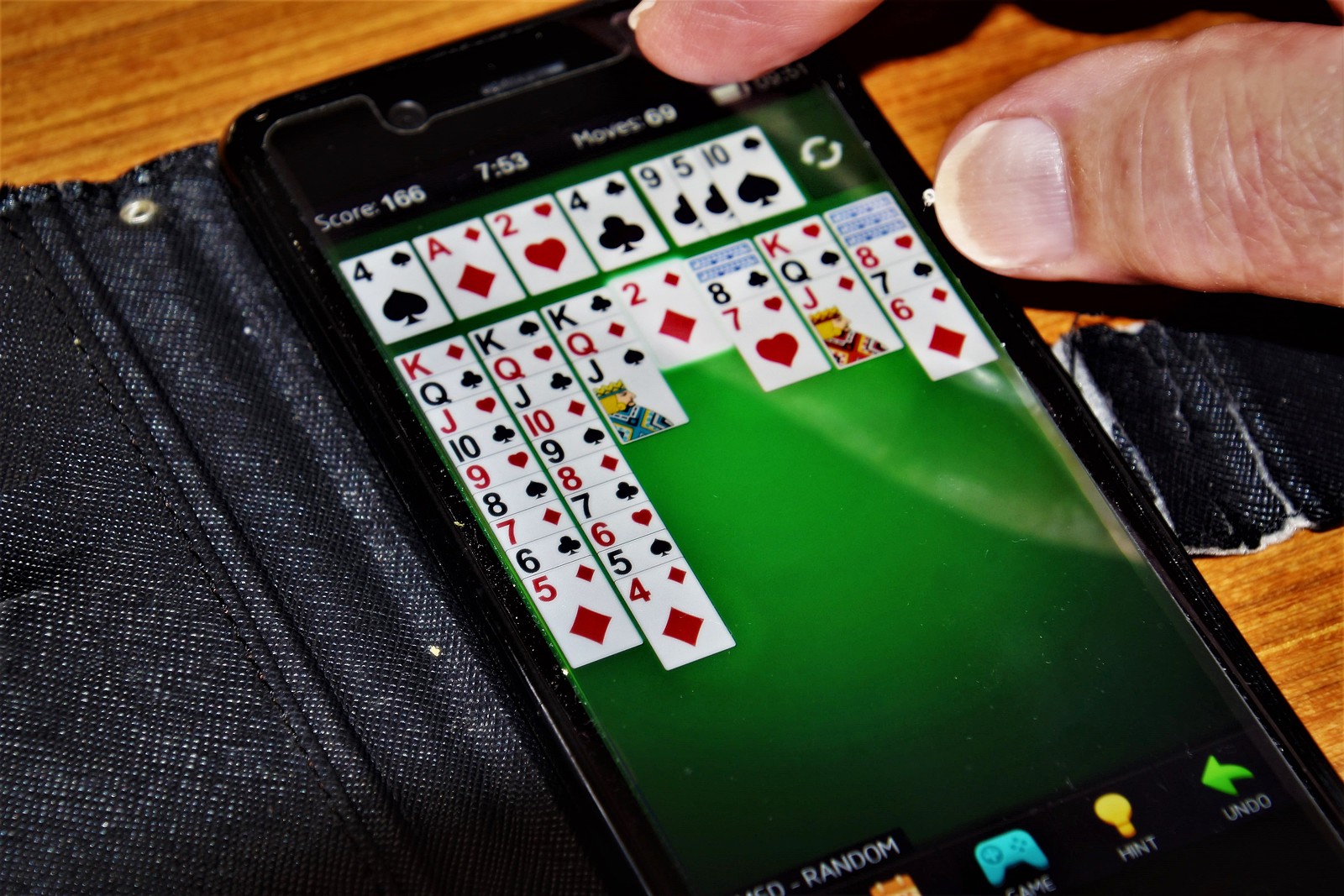In this image, we see a close-up of a smartphone screen displaying a Solitaire game in progress. The screen reveals seven columns of cards: the first three columns begin with a King and descend. One column descends from a King to a Five, another from a King to a Four, and the third from a King to a Jack. The top cards of the remaining four columns are the Two of Diamonds, Seven of Hearts, Jack of Diamonds, and Six of Diamonds, respectively.

At the top of the screen, there are four foundation piles for aces and ascending numbers. The spades foundation has a high card of Four, the diamonds foundation shows only an Ace, the hearts foundation has a high card of Two, and the clubs foundation also displays a high card of Four. The draw pile shows a sequence with the top card being the Ten of Spades, followed by the Five of Clubs, and the Nine of Clubs.

The game's interface shows a score of 160, a time of 7:53, and 69 moves made. The game is set against a green background, and several control buttons are visible at the bottom of the screen. The phone is encased in a cloth cover that has a black and white rough denim appearance. The image captures the thumb and the tip of the forefinger of a man who is holding the phone and actively playing the Solitaire game.